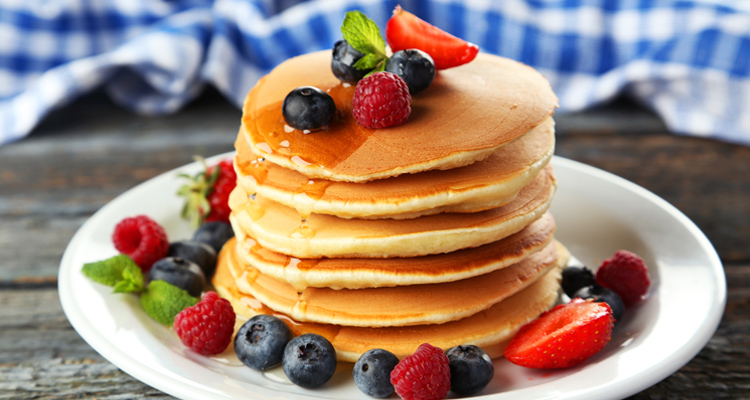This image features a mouth-watering stack of six medium-sized, fluffy pancakes arranged on a white plate. The pancakes are adorned with a medley of fresh berries, including strawberries, raspberries, and blueberries, adding a burst of color and flavor. A few sprigs of green garnish, likely mint leaves, are scattered artfully for aesthetic appeal. A light drizzle of syrup cascades down the front of the pancakes, enhancing their appetizing appearance. Surrounding the stack on the plate are additional berries and mint leaves, creating a visually pleasing presentation. The plate rests on a dark wooden table, with a blurred blue and white checkered tablecloth in the background, contributing to a cozy and inviting atmosphere.